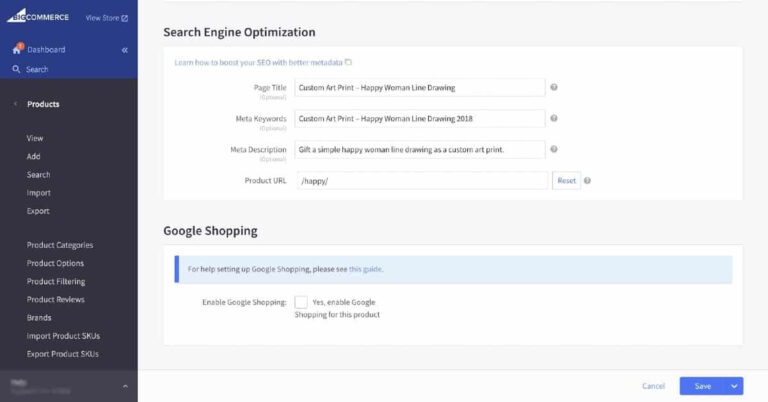The image shows a detailed interface related to search engine optimization (SEO) for an e-commerce platform. At the top, there is a heading that reads "Search Engine Optimization." Below this, there is a subheading that says, "Learn how to boost your SEO with better metadata." 

The interface includes several metadata fields:

- **Page Title:** Custom Art Print | Happy Woman Line Drawing
- **Meta Keywords:** Custom Art Print, Happy Woman Line Drawing, 2018
- **Meta Description:** The description text is partially blurry, but it starts with "Get a simple happy woman..." 

Additionally, there is a section about setting up Google Shopping, which includes the message: "For help setting up Google Shopping, please see this guide." There are options to enable Google Shopping for the product, with a selection toggle labeled "Enable Google Shopping" set to "Yes."

On the left sidebar, there are multiple navigation options for managing the online store, including:
- BigCommerce
- View Store
- Dashboard
- Search Products
- View, Add, Search, Import, Export Products
- Product Category
- Product Option
- Product Filtering
- Product Reviews
- Brand
- Import Product SKUs
- Export Product SKUs

This interface appears to provide comprehensive tools for optimizing products for search engines and integrating with Google Shopping to enhance the visibility and sales of the listed products.